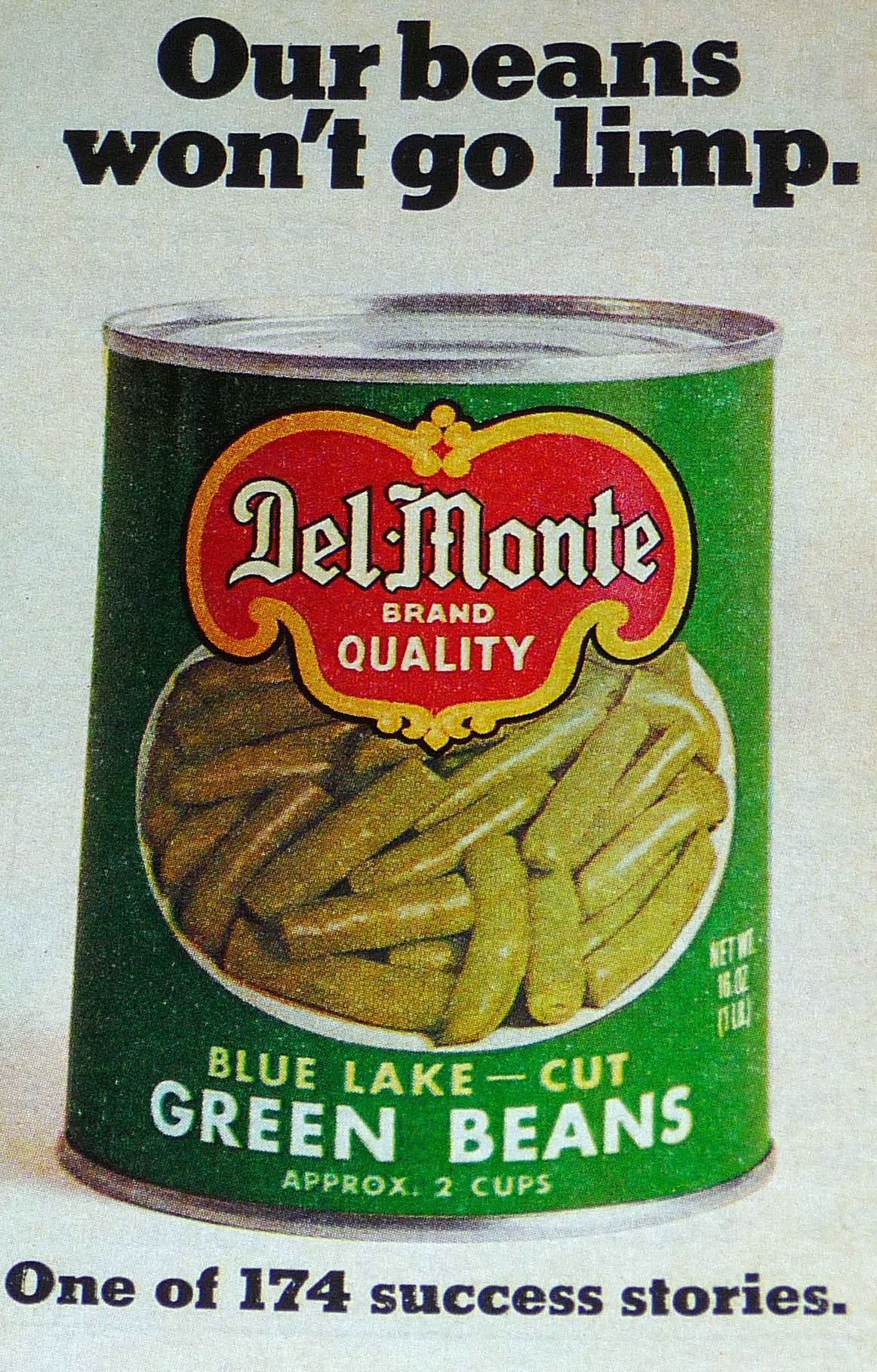The image is a magazine advertisement for Del Monte Green Beans set against a cream-colored background. At the top, bold text states, "Our beans won't go limp." Below this headline is a close-up of a green can of Del Monte Blue Lake Cut Green Beans. The can features a red crest-shaped Del Monte logo with the words "Brand Quality" underneath in white letters. Within the red crest, there's a circular image displaying the green beans themselves, which are depicted in a white bowl. The can’s label, which is lighter green than the actual beans, also includes the text "Blue Lake Cut," "Green Beans," and "Approximately Two Cups." At the bottom of the image, in black text, it reads, "One of 174 success stories," signifying the brand’s pride and confidence in their product.